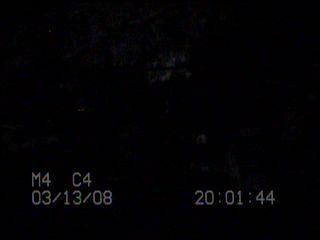The image is a small rectangular photograph, likely taken from a surveillance or security camera, characterized by its predominantly black background. At first glance, it appears as if there is nothing visible due to the overwhelming darkness, but upon closer inspection, a faintly lighter shape, possibly resembling a tree, is discernible in the center. This image, which appears to be a vintage or dated screenshot, displays white digital text at the bottom. On the lower left, the text reads "M4C4" in a bold typeface, followed by the date "03/13/08," indicating it was taken on March 13, 2008. In the lower right corner, a timestamp of "20:01:44" is visible, suggesting the image was captured at 8:01 PM and 44 seconds.